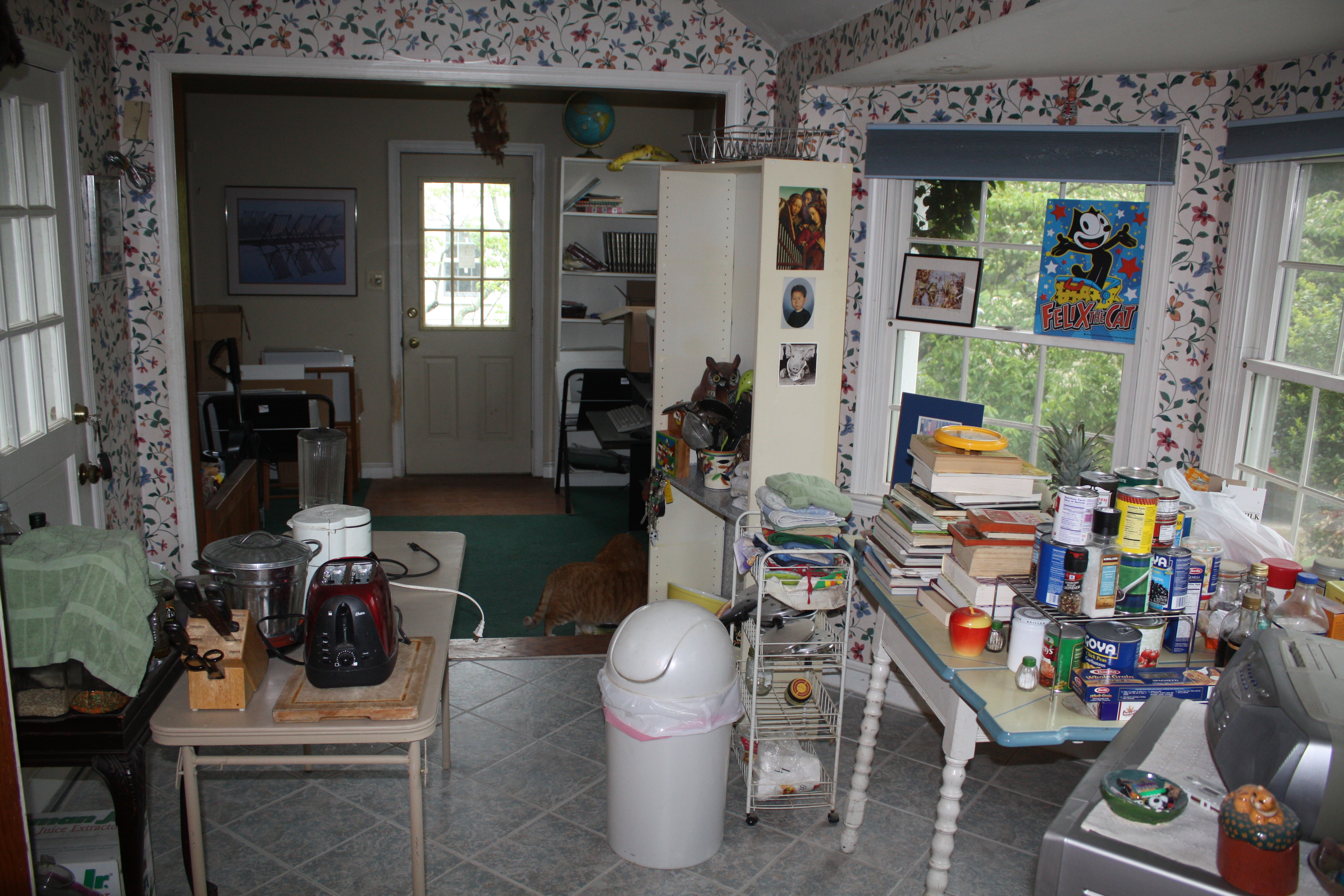This photograph captures a chaotic kitchen viewed from an elevated doorway perspective. The room features a hexagonal bump-out and walls decorated with pink, blue, and green floral wallpaper against a white background. The left-hand side of the room holds a tan folding table cluttered with a knife block containing black-handled knives, a black and silver toaster, a rice cooker, and a white coffee pot. A cherry-style queen-end table stands behind it, topped with an animal cage draped in a green towel, and is adjacent to an exterior wooden door with a solid bottom and three-over-three glass panels on top.

In the center of the kitchen is a white plastic garbage can with a flip-top lid, next to a white rolling wire cart brimming with assorted kitchen items, books, and towels. A large farmhouse table painted white with a blue trim dominates the space, laden with canned goods stacked three cans high, a collection of oil bottles, and an assortment of cookbooks.

The background reveals an adjoining room with green carpet, further disarray marked by folding chairs piled with items, a bookcase spilling over with books, and another wooden door matching the exterior one. A poster featuring a black and white cartoon cat, Crazy Cat, set against a blue background, decorates one of the back windows, adding a whimsical touch to the scene.